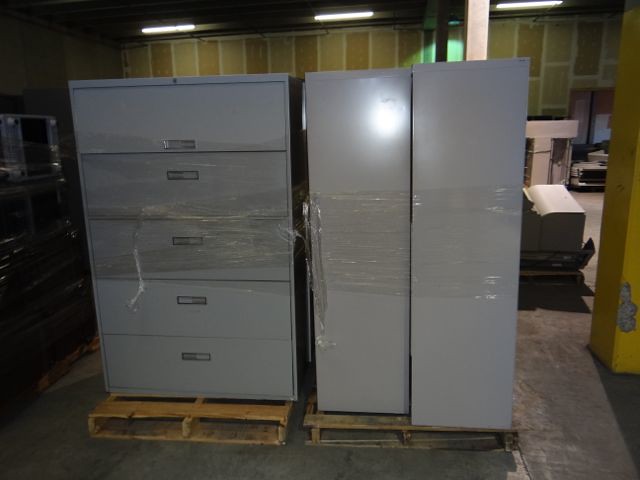The image captures an indoor setting, likely a warehouse or abandoned office space, characterized by a gray concrete floor and dim lighting. At the forefront, there are three tall filing cabinets, each with five drawers and a slot for a key at the top. These gray cabinets are wrapped in clear shrink wrap around the middle and are placed on tan wooden pallets. To the left, additional office furniture, also wrapped in shrink wrap, is visible, though the area is quite dark. The scene is illuminated by bright white fluorescent lights evenly spaced at the ceiling. The background wall features a patchwork of gray, green, and cream rectangles separated by white panels, and on the right stands a tall yellow concrete pillar with a chunk missing at its base. Scattered around are empty boxes and other miscellaneous furniture pieces, emphasizing the disorganized, transitional state of the space.